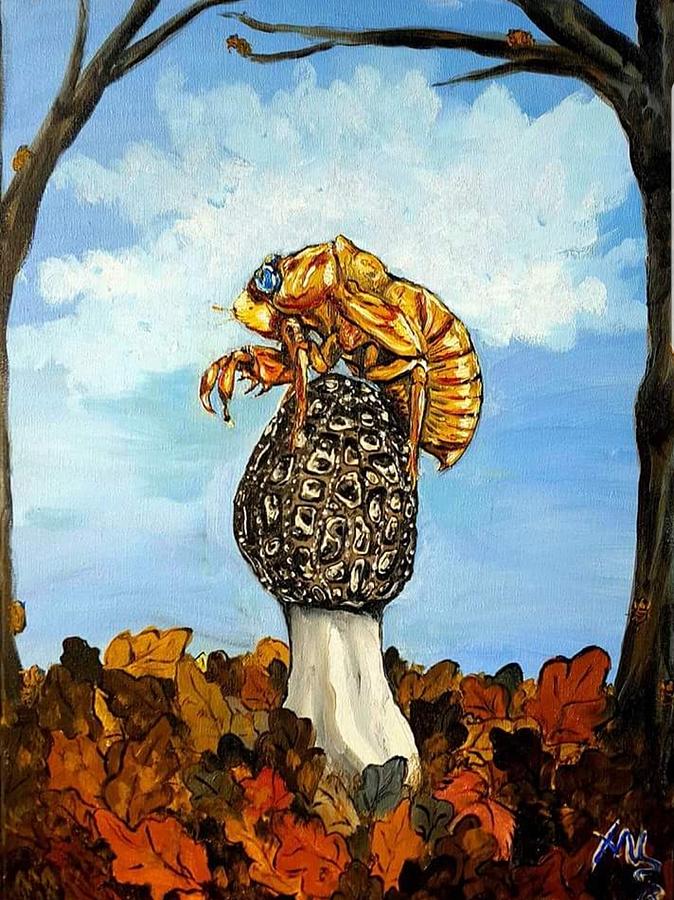This detailed oil painting captures a surreal scene centered around a large mushroom with a white stem and a dark gray, intricately patterned cap. Perched atop the mushroom is an ornate, golden insect that resembles a cicada. This insect, detailed with copper accents and a distinctive blue eye, faces left, adding an intriguing focal point to the artwork.

At the base of the mushroom, autumn leaves in shades of red, orange, and yellow blanket the ground, evoking the richness of fall. On the left and right of the image, bare trees with scattered leaves extend their limbs towards each other, forming an arch-like frame around the central elements. The background features a bright blue sky adorned with a single, large puffy white cloud, providing a stunning contrast to the warm, earthy tones below.

The signature of the artist appears in dark blue, outlined by white, in the bottom right corner of the painting. The visible brush strokes in the sky add texture and depth to this captivating and complex scene.